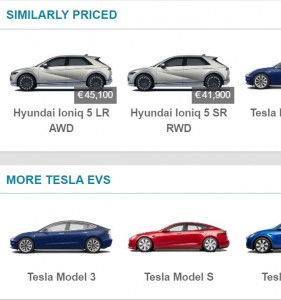This section of a web page features a comparative display of electric vehicles, predominantly showcasing models from Hyundai and Tesla. The background of the display is uniformly white, emphasizing the vehicle images or highly realistic drawings against the clean backdrop.

At the top of the section, the phrase "Similarly Priced" is prominently displayed in blue font. Immediately below, three specific car models are presented from left to right:
1. **Hyundai Ioniq 5 LR ADR**: This gray SUV is priced at €45,100.
2. **Hyundai Ioniq 5 SR RWD**: Another gray vehicle priced at €41,900.
3. **Tesla (Model Unspecified)**: Only a partial view of this car is visible, displaying the front part in blue, and the name is cut off so only "Tesla" is legible.

Below these vehicle images is a gray border, separating the section with more details about additional Tesla electric vehicles, indicated by the blue text "More Tesla EVs".

Underneath this header, three Tesla models are showcased:
1. **Tesla Model 3 (Blue)**: An image of the full blue car is shown, though no price is listed.
2. **Tesla Model S (Red)**: The image depicts this sporty, red-colored car.
3. **Unspecified Tesla Model**: Only part of this blue vehicle is visible, revealing just the front section and part of the windshield. The text displayed cuts off after "TES" but it is identifiable as a Tesla.

Overall, this segment of the webpage provides a comparative look at select Hyundai and Tesla electric vehicles, highlighting their prices and basic visual features.